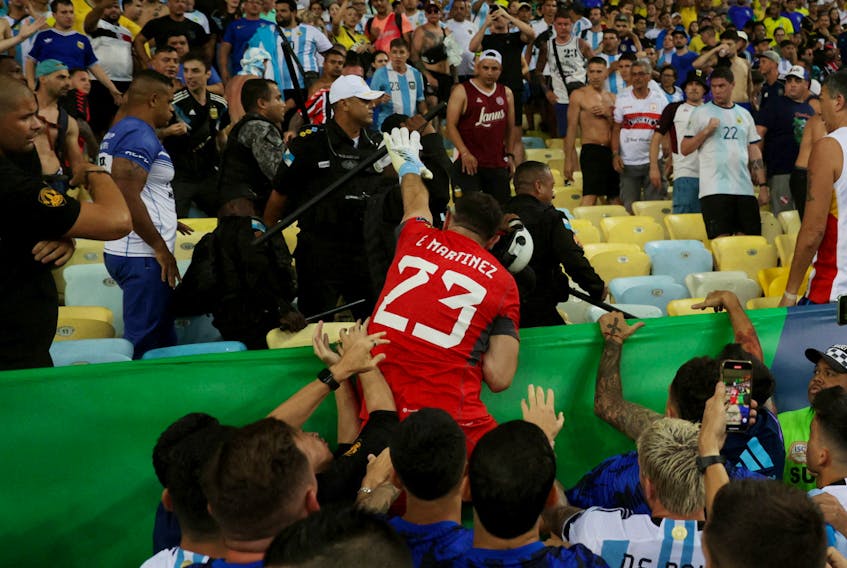In this chaotic scene captured at a soccer match, fans and players alike are embroiled in commotion. The focal point of the image is a player in a red jersey with the name "Martinez" and the number 23 emblazoned on the back. He is wearing a white glove and appears to be reaching up towards the stands where security personnel, identifiable by a nightstick, are present. The fans, some shirtless and others in jerseys, are packed into the stadium’s blue and yellow seats, all intently focused on a specific area, suggesting either a celebratory moment turned chaotic or an altercation. Martinez seems to be climbing a wall, possibly to interact with the crowd or address the disturbance. Surrounding him, teammates in Adidas-branded jerseys also seem engaged, either assisting him or reaching towards the stands. The atmosphere is electrified, with some fans in the background documenting the event on their phones.